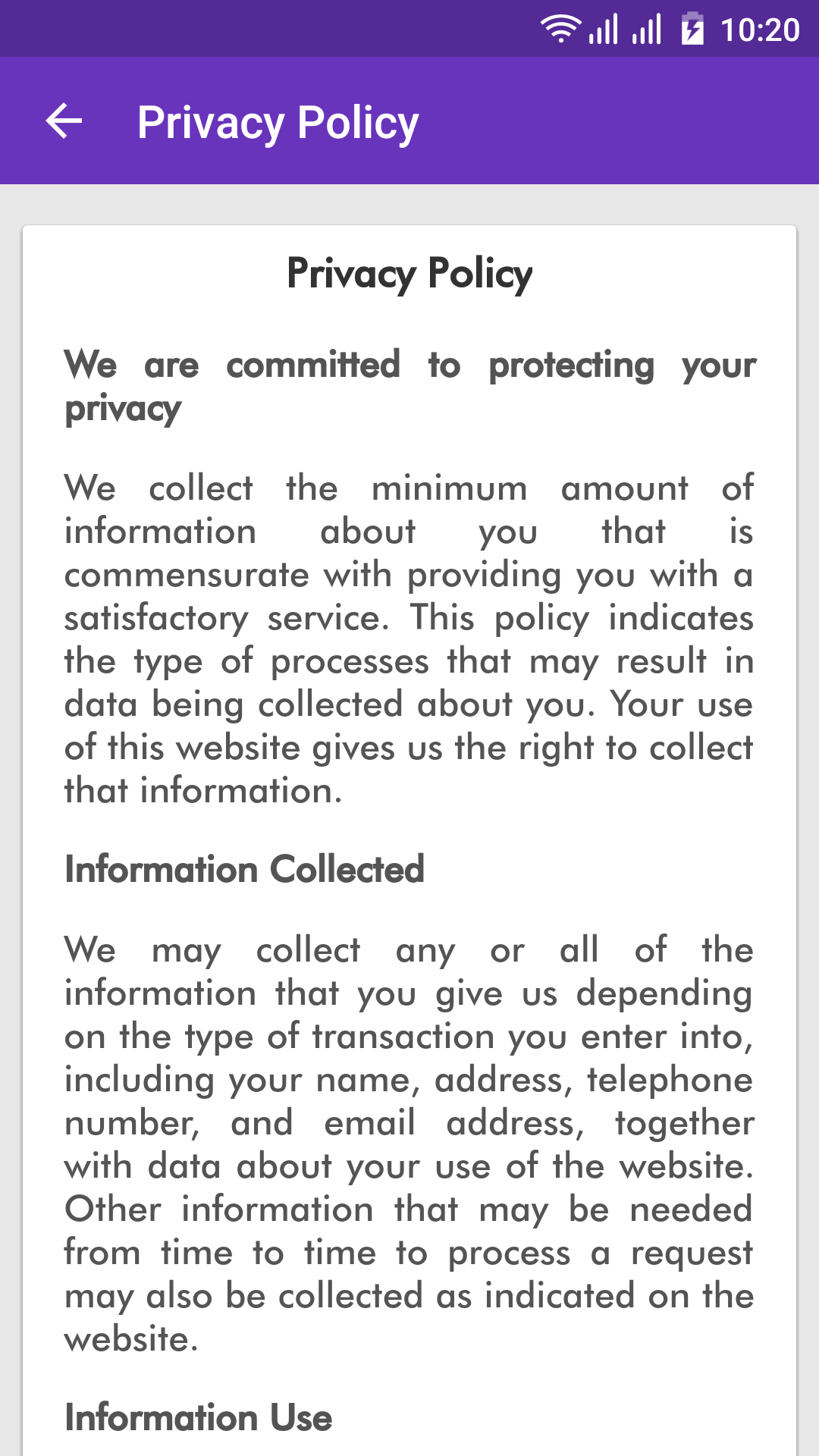The image displayed on the smartphone screen captures the privacy policy section of a website. At the top of the screen, various status icons are visible: the Wi-Fi signal strength, a fully charged battery indicated by a lightning bolt, and the current time shown as 10:20 AM. Just below these icons, a prominent purple banner with white text reads "Privacy Policy" and features a white arrow pointing to the left, possibly indicating a navigation option. 

As one scrolls down, the content of the privacy policy is visible. It begins with a statement of commitment to user privacy, emphasizing the collection of minimal information necessary to provide satisfactory service. The policy outlines the types of data that may be collected, including personal details such as name, address, telephone number, and email, as well as data regarding website usage. Additional information may also be collected as needed to process specific requests, as indicated on the site. The section starts with a clear header "Privacy Policy" followed by the statement: "We are committed to protecting your privacy. We collect the minimum amount of information about you that is commensurate with providing you with a satisfactory service. This policy indicates the type of processes that will result in data being collected by you. Your use of this website gives us the right to collect that information and information collected. We may collect any or all of the information that you give us depending on the type of transaction you enter, including your name, address, telephone number and email address together with data about your use of the websites. Other information that may be needed from time to time to process a request may also be collected as indicated on the website." This introduction is followed by the heading "Information Use," which likely elaborates further on how the collected data will be utilized.